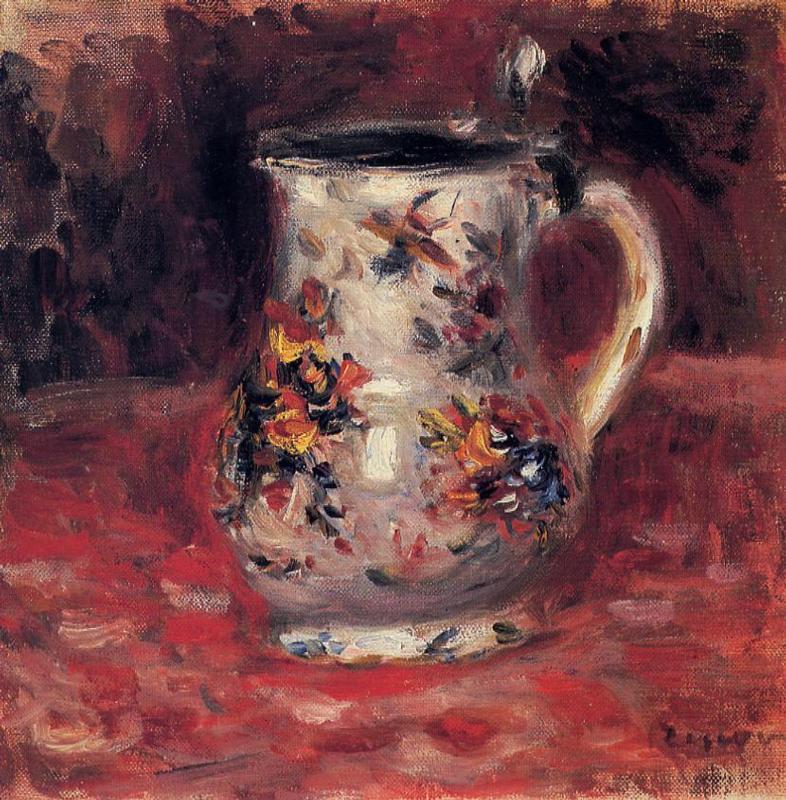The image is an abstract, hand-painted drawing depicting a white jar with a curved handle on the right side, sitting centrally on a table. The jar features intricate flower patterns in red, orange, and blue and has a distinctive shape with a narrower top and base and a wider body. The table beneath the jar is predominantly red with hints of black and white patches, occupying the bottom half of the painting. The background above the table is a mix of dark colors, primarily black with touches of red, showcasing the contrast and depth typical of an oil painting. The artist's signature is subtly placed at the bottom right, though it is not clearly legible. The overall composition and color palette create a richly textured, visually compelling piece.